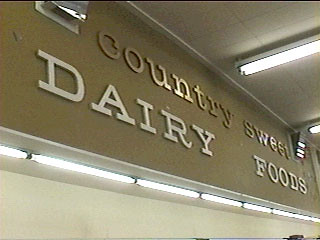This indoor photograph captures a section of a grocery store, specifically the dairy aisle, from a diagonal angle looking up towards a banner mounted on a green-hued wall. The banner, featuring the text "country sweet" in lowercase letters at the top and "DAIRY FOODS" in all capital letters underneath, is prominently displayed. The letters are depicted in a lighter green or brownish hue against a muted brown or green backdrop. Above the banner, to the upper left, the ceiling is visible, showcasing a beige tone with a grid of rectangles formed by black lines. Part of a thin fluorescent light tube is seen extending perpendicularly from the right side of the ceiling. Additional fluorescent light tubes hang slightly diagonally under the banner on the wall, enhancing the illumination of the signage. Below the banner, the wall transitions to a white color. The overall image is well-lit and sharply focused, drawing clear attention to the "Country Sweet Dairy Foods" sign, though no actual groceries are visible in the frame.